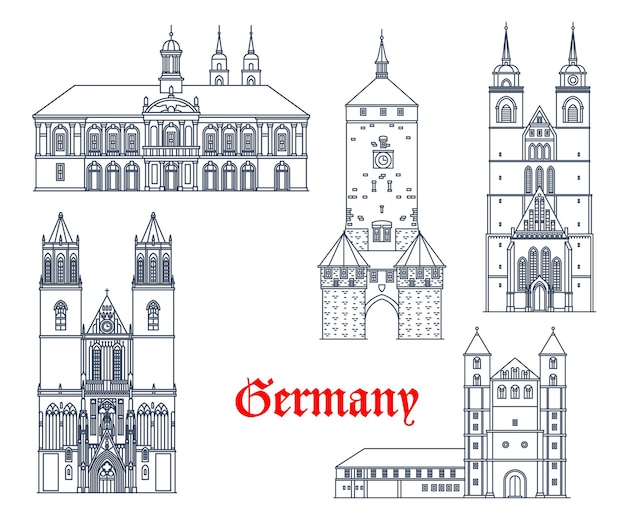The image is a detailed, black-and-white line art illustration featuring architectural renderings of various buildings in Germany. It has a white background with the word "Germany" prominently displayed near the bottom center in a gothic red typeface. The image has five distinct architectural illustrations arranged with three across the top and two along the bottom.

On the top left, there's a wide, palatial structure with a central tower and a two-tiered porch featuring arched windows. This building also includes two additional smaller towers. The upper middle centerpiece showcases a tall, single tower crowned with a spiral-shaped roof, flanked by two smaller towers with an arched entry in between. On the top right, a large vertical structure features two side towers and a central gable rising four stories high.

At the bottom left, another building resembles the upper middle structure but includes a two-story gable in the center and towers to the left and right. The bottom right structure displays a combination of two towers, a central gable area, and an adjoining shorter building on the left side. The entire composition emphasizes intricate architectural details with blue-pen outlines and white bodies, creating a cohesive and striking visual ensemble.